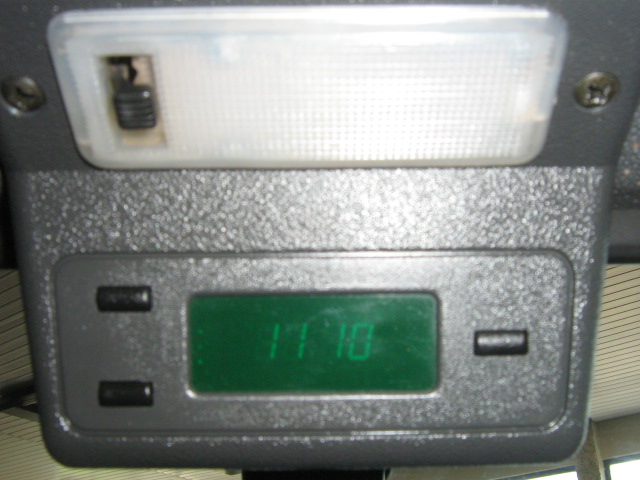This photograph captures a digital clock embedded in a textured, gray plastic mount, reminiscent of what might be found on the dashboard of a car, or mounted in an aircraft or boat. The clock itself features a green LCD screen displaying the time "11:10". Surrounding the screen, the device's faceplate is anchored by Phillips screws on either side. Directly above the clock display, there is a white rectangular light encased in a clear plastic cover. This light is accompanied by a sliding black switch on its left side. The light fixture has a slightly square appearance. On the left side of the clock's faceplate are two black lozenge-shaped buttons, positioned one above the other, while on the right side there is a single matching button. In the background, a window frame with an upright bar is partially visible, enhancing the scene's depth and context.